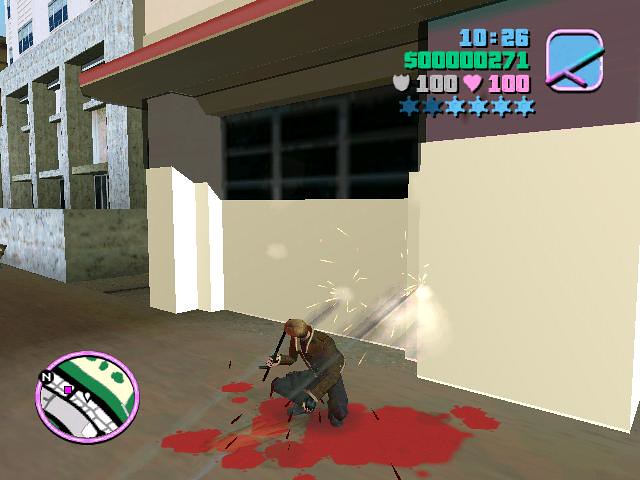In this still image from what appears to be the video game Grand Theft Auto, we are presented with a detailed and intense scene. A man, possibly trying to dodge bullets, is kneeling or bending down on a ground that looks brown or cement-like. He is dripping blood, which is clearly splattered on the ground. He wears a long brown jacket and black pants, suggesting he is either injured or engaged in combat, possibly holding a weapon like a gun or a sword. 

In the top right corner of the screen, various game indicators are visible. The time reads 10:26 in blue, and beside it, $0000271 in green indicates possibly the character's cash. A badge with '100' in light gray and a pink heart with '100' may show his health or shield status. Additionally, there are six stars, with the first two being dark blue and the next four light blue, which could signify a wanted level or achievement status.

On the left side of the screen, we can see a pink circle with green, gray, and white lettering, including the letter 'N' inside a black circle. The background features a brown terrain with a structured environment. There are detailed buildings: an off-white one with darker gray columns and red accents, and another gray cement building with vertical and horizontal strips. There's also a pink square with a line forming a V shape in pink, transitioning to light blue, adding to the game's vibrant and chaotic ambiance.